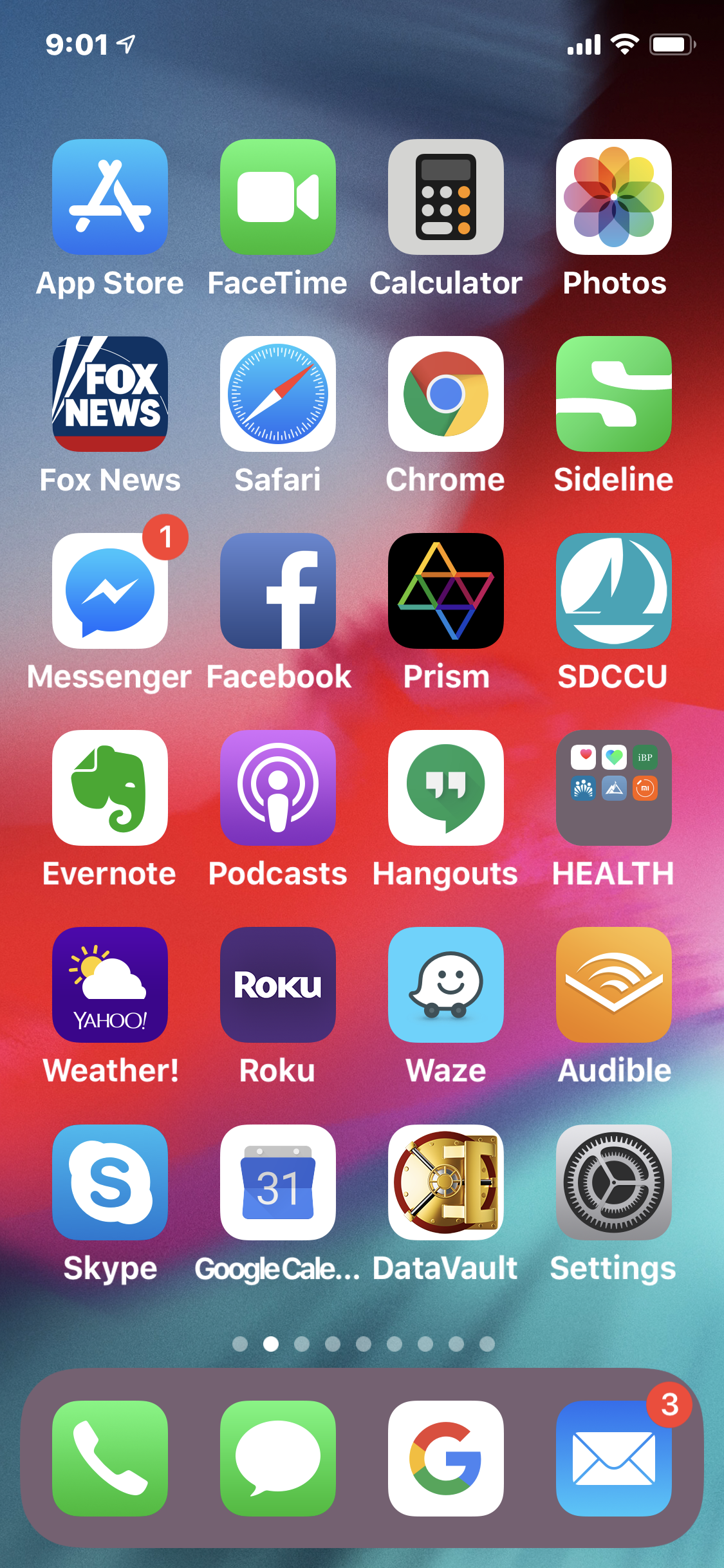The image showcases the home screen of an iPhone, intricately adorned with a myriad of app icons arranged over a gradient background transitioning from blue at the top, through purple and pink, to red, and finally to dark gray at the bottom. In the upper left corner, the time is displayed as 9:01, accompanied by icons indicating signal strength, Wi-Fi connectivity, and battery life.

The dock at the bottom of the screen features four primary app icons: Phone, Messages, Google, and Mail. Above the dock, various app icons are scattered across the colorful background, including essentials like App Store, FaceTime, Calculator, Photos, Fox News, Safari, Chrome, Sideline, Messenger, Facebook, Prism, SDCCU, Evernote, Podcasts, Hangouts, Health, Weather, Roku, Waze, Audible, Skype, Google Calendar, Data Vault, and Settings.

Three notable red-colored icons stand out against the blue backdrop of the screen, enhancing the visual appeal and organization of the apps. The carefully arranged applications and detailed backdrop create a cohesive yet vivid design for the iPhone's home screen.